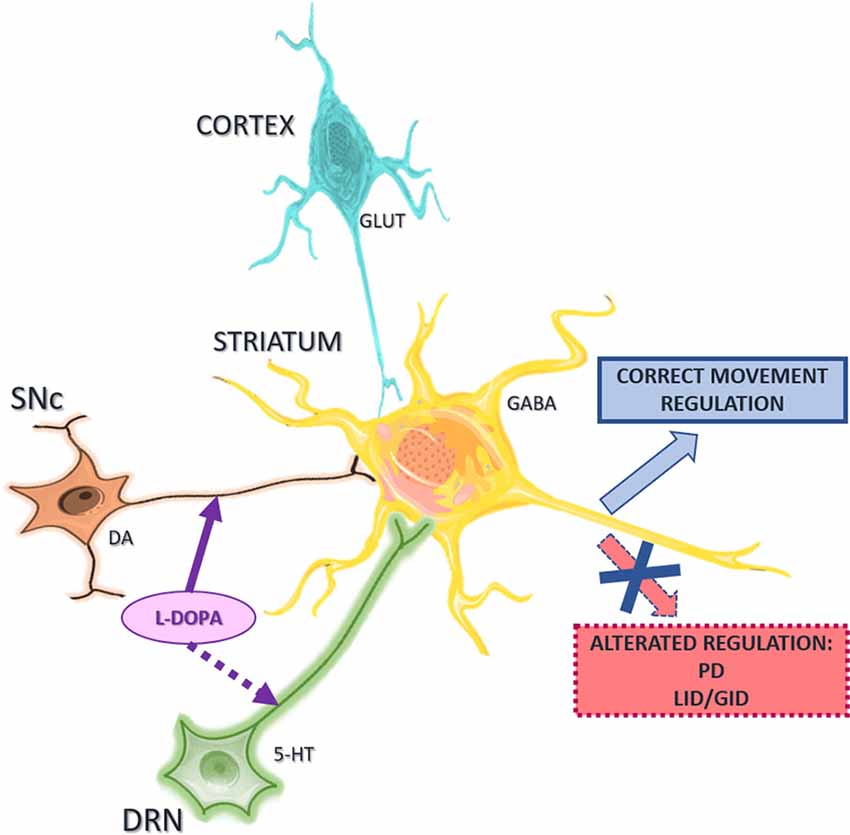The image is a detailed and colorful diagram on a white background, illustrating various aspects of brain function. Key components include a blue-labeled cortex at the top, which connects to a yellow-highlighted striatum in the center. From the striatum, pathways lead down to the green-labeled DRN and the star-shaped NSNC. The diagram prominently features multiple labels, such as GABA, GLUT, 5-HT, and L-DOPA, with arrows indicating regulatory pathways and connections. For instance, a blue arrow from the GABA label points to a section labeled "Correct Movement Regulation." Additionally, a clay-colored label with dark text states "Altered Regulation, PD, LID/GID." The diagram is intricately designed with shades of teal, blue, peach, green, and yellow to distinguish the various components and their interconnections, providing a visual representation of how these elements contribute to brain function and regulation.